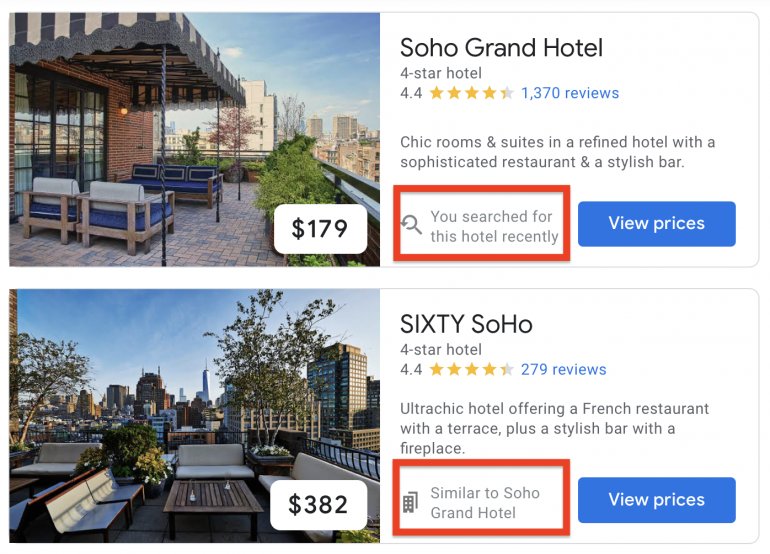The image features two stacked photographs of urban outdoor scenes. The top image displays a cozy seating area with blue-cushioned chairs under an awning, surrounded by small bushes and a railing, with buildings visible in the background. This image includes a price tag of $179. It is labeled as the Soho Grand Hotel, a 4-star establishment with a rating of 4.4 based on 1,370 reviews, boasting chic rooms and suites, a sophisticated restaurant, and a stylish bar. The text also indicates that this hotel was searched for recently, highlighted by a red box.

The bottom image exhibits a similar ambiance but lacks an awning and doesn't show the connecting building. The seating area remains, but with a price tag of $382. This image is captioned as 60 Soho, another 4-star hotel with a rating of 4.4 from 279 reviews. Similarly, a red box highlights that this hotel is comparable to Soho Grand Hotel.